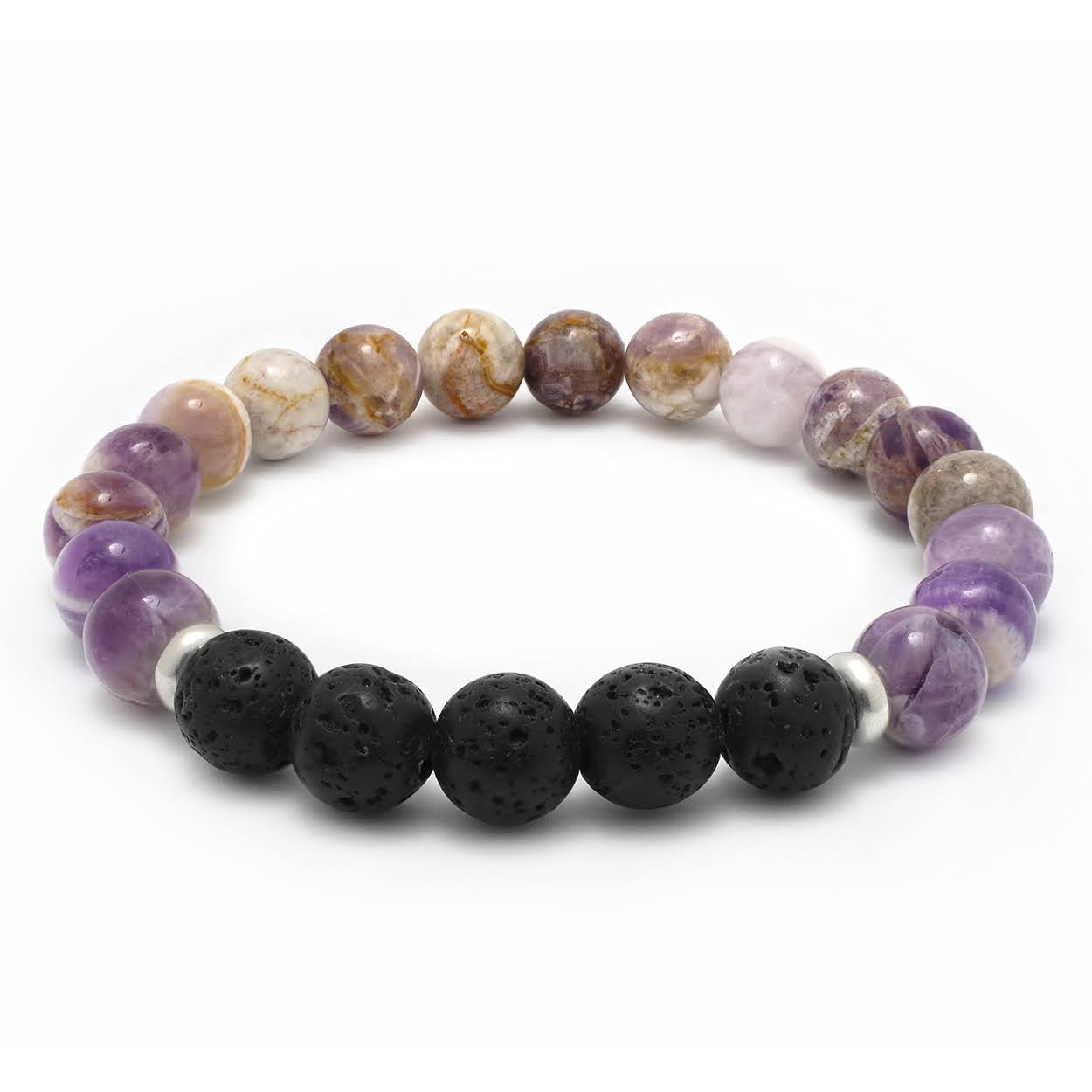This is a detailed close-up photograph or a highly realistic artist's rendition of a wristband or necklace, composed of 22 beads arranged in a perfect circle against a stark white background, which accentuates the vivid colors and textures of the beads. The wristband starts with five jet-black beads in the foreground, each with small pitted holes or markings. These black beads are flanked by smaller silver-colored stoppers to separate them from the rest. Beyond these, there are eight distinctive purple, amethyst-like beads scattered throughout the circle. Completing the circle are a variety of other stones: some are a combined white, gold, and lilac marble pattern, while others display mottled gray and clear tones. Each bead, whether black, purple, or otherwise, is oval-shaped, contributing to the harmonious yet varied aesthetic of the piece. The entire setup casts a subtle shadow on the white surface beneath it, adding depth to the minimalist composition.